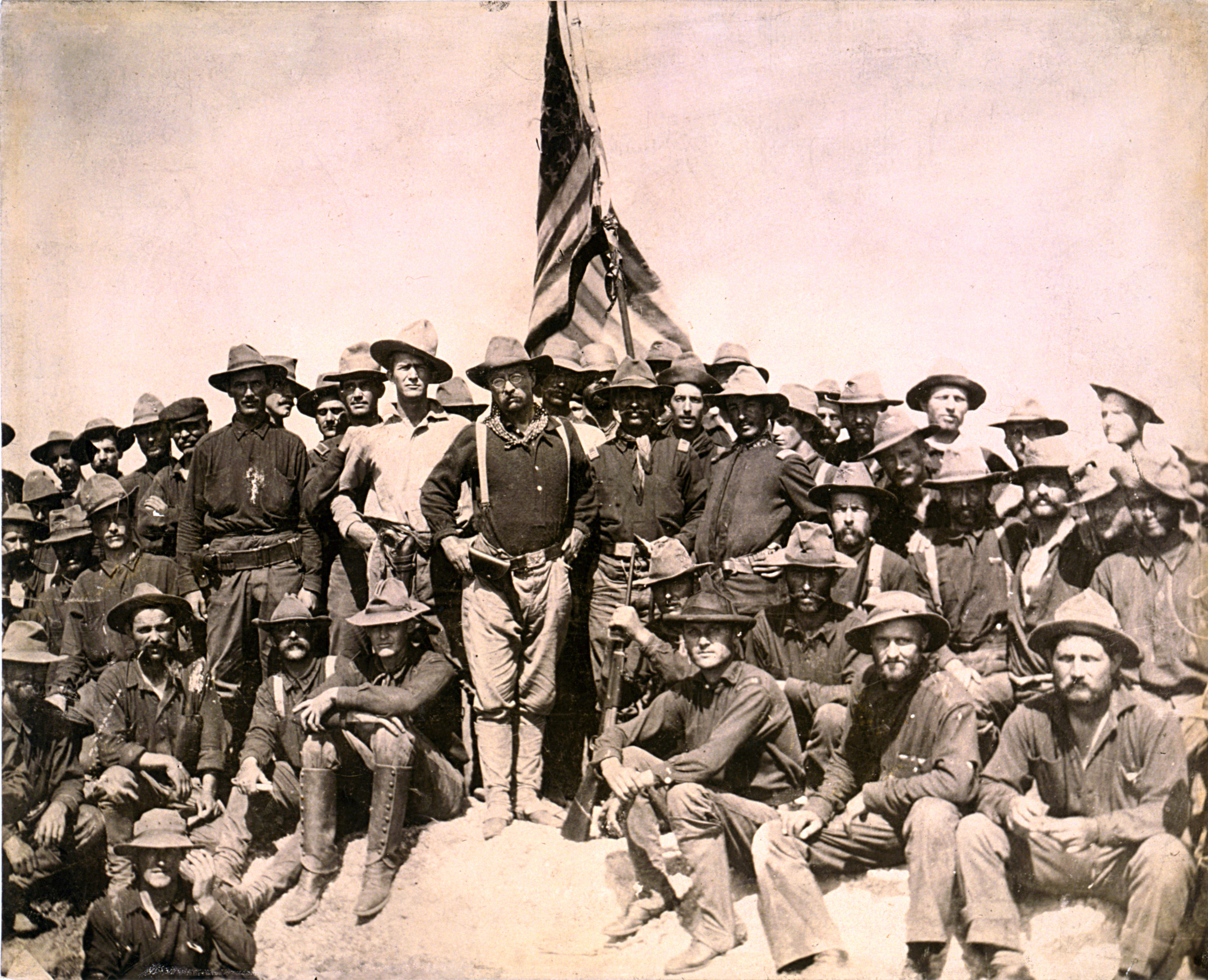This black and white photograph features a historic image of Theodore Roosevelt and his Rough Riders. The sky has a grayish, whitish hue, suggesting it is daytime. An American flag prominently rises in the upper center portion of the image, held by the group of men gathered beneath it. These men, who are either soldiers or cowboys, wear hats resembling cowboy hats, and are adorned in dark-colored long-sleeve shirts and long pants. Some wear boots and suspenders, and they are arranged in several rows: a front row where men are seated and two or more rows of men standing behind them. The photograph’s overall appearance shows signs of color distortion over time, giving it a subtle pinkish tinge, unique to old photographs. Most of the men are facing forward, many with slight head tilts, capturing a solemn and unified stance.